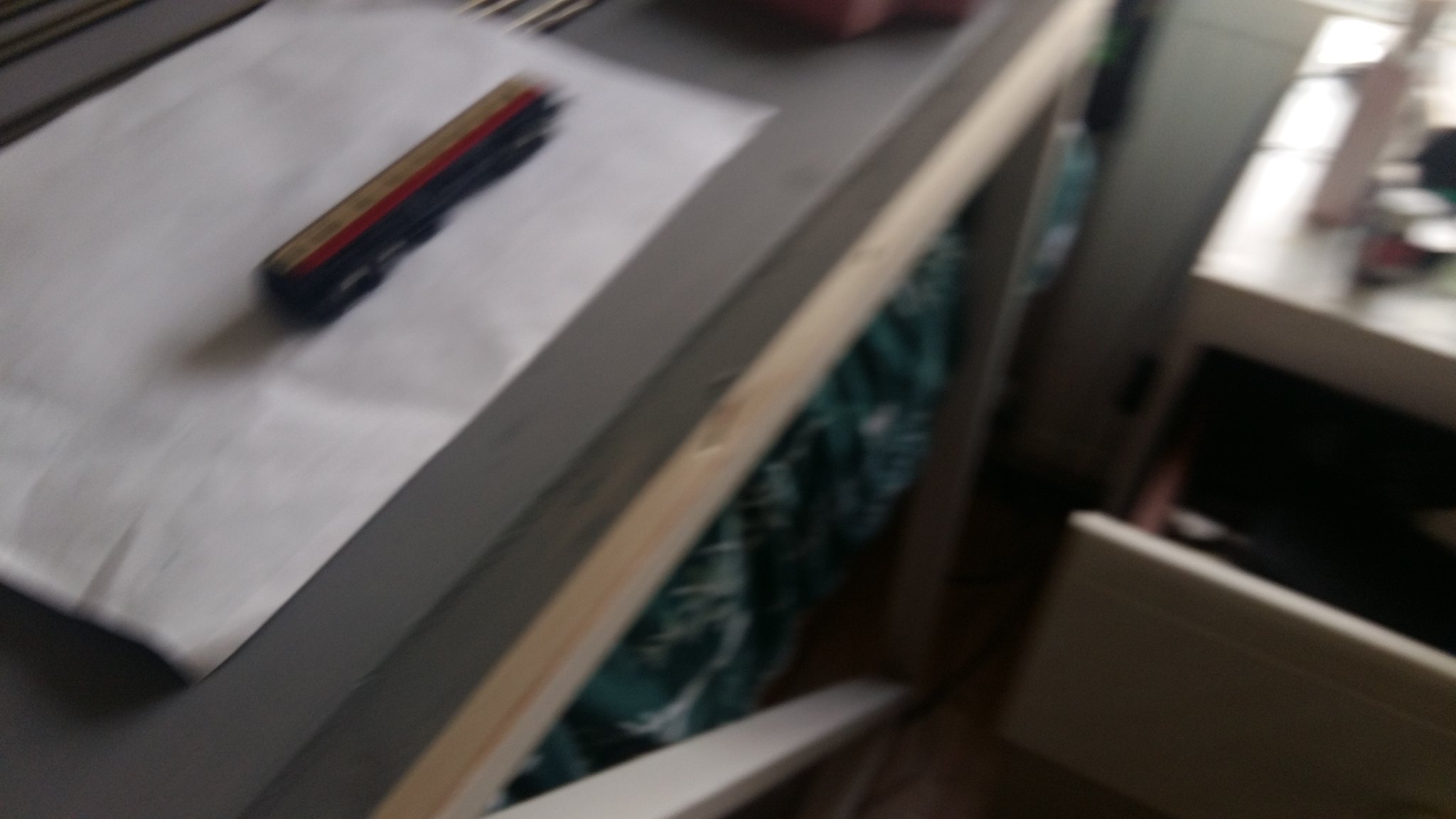This image captures a slightly blurry scene of a room featuring a variety of furniture and objects. On the left side, there's a gray platform or table with metal rods for support and a wooden trim. The top surface holds a white sheet, and on top of it, a distinct blue object that resembles a box cutter, with a red and brown strip running along its length. There is also a weight placed on this white sheet. Under the platform, some bluish sheets are visible. To the right, there's a white nightstand with a drawer that is partly open, revealing a dark, black interior. The nightstand's top surface hosts several items, including a white bottle with a pump and some small white canisters, one of which is red with black outlines.